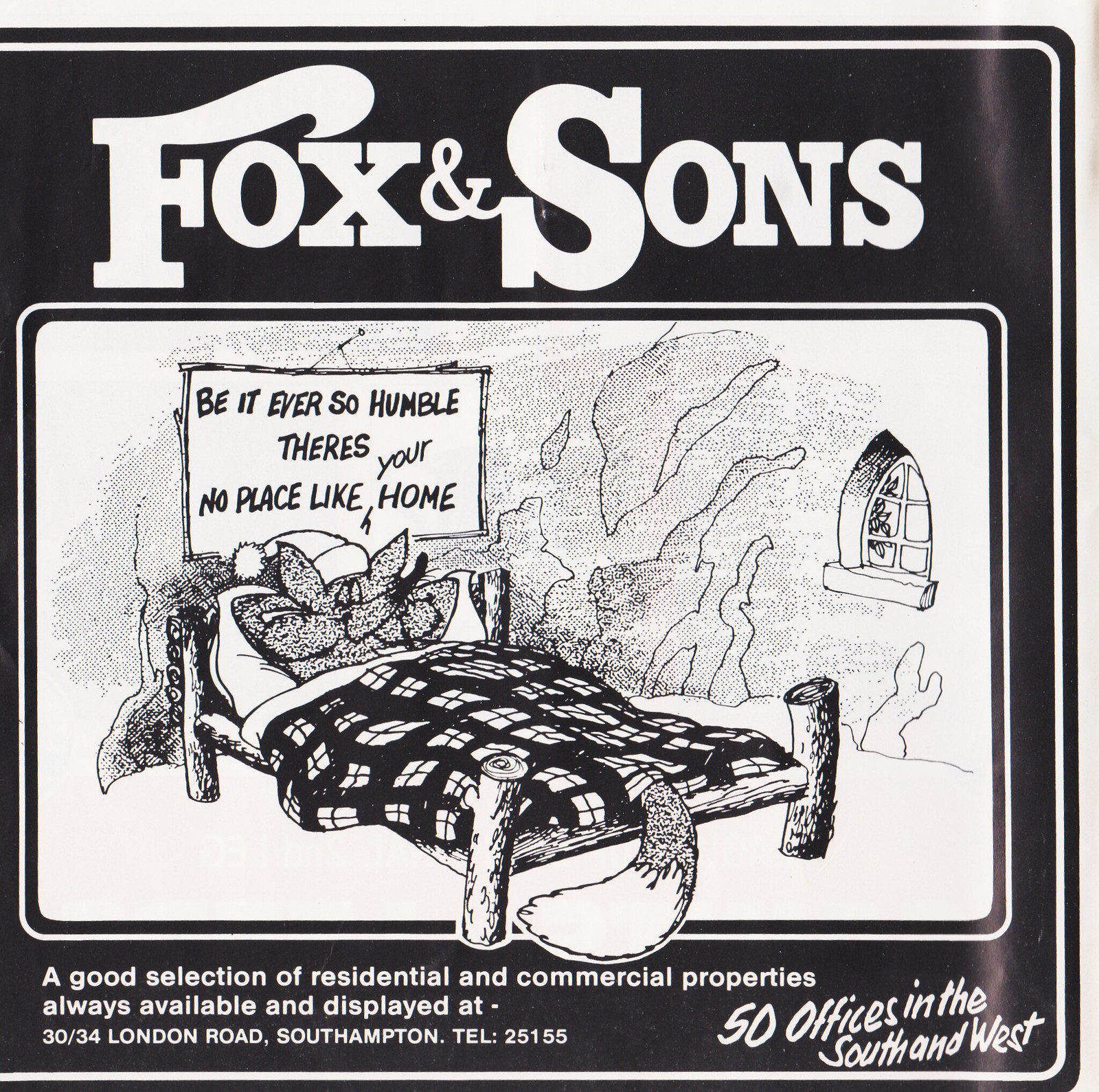This black and white advertisement for Fox and Sons features a central cartoon illustration of a fox lying comfortably in a rustic log bed, covered with a black and white plaid blanket, its tail peeking out from the bottom. The fox wears a sleeping cap with a tassel, and above its head hangs a sign reading "Be ever so humble, there's no place like your home," with "your" handwritten between "like" and "home." The bed is set inside what appears to be a cave, complete with an arched window. Below the image, the ad mentions, "A good selection of residential and commercial properties, always available and displayed at 30-34 London Road, Southampton." The telephone number listed is 25155, and it notes that Fox and Sons operate in "50 offices in the South and West."